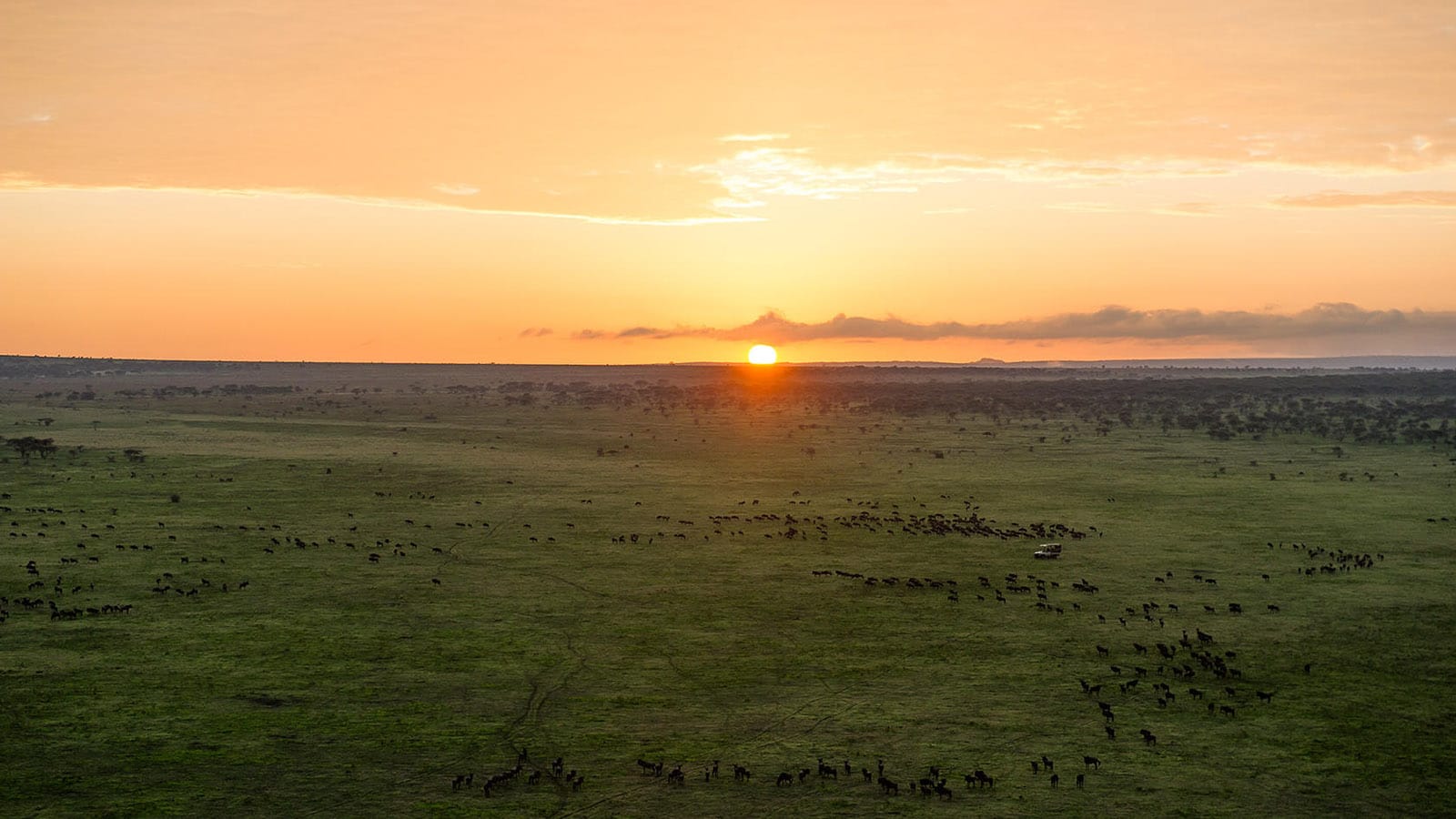In the very center of the image, there is a striking scene of the sun positioned low on the horizon, either rising or setting, suggesting it is either early morning or late afternoon. The sky is a dramatic palette of orange hues, interspersed with white and dark gray clouds moving in from the right. Below the sun lies a vast expanse of lush green grass, interspersed with patches of weeds, dominating the lower half of the image. Scattered throughout this verdant field are groups of animals, dark in color, with their exact species indistinct, adding a dynamic element to the scene. These animals appear to be part of a caravan that stretches from the lower border of the picture towards the right center, and then veers back towards the left center. Amongst them, a truck positioned in the central green area seems to be herding the animals, orchestrating their movement across the grasslands. The overall composition captures a harmonious yet bustling moment of life beneath a captivating sky.